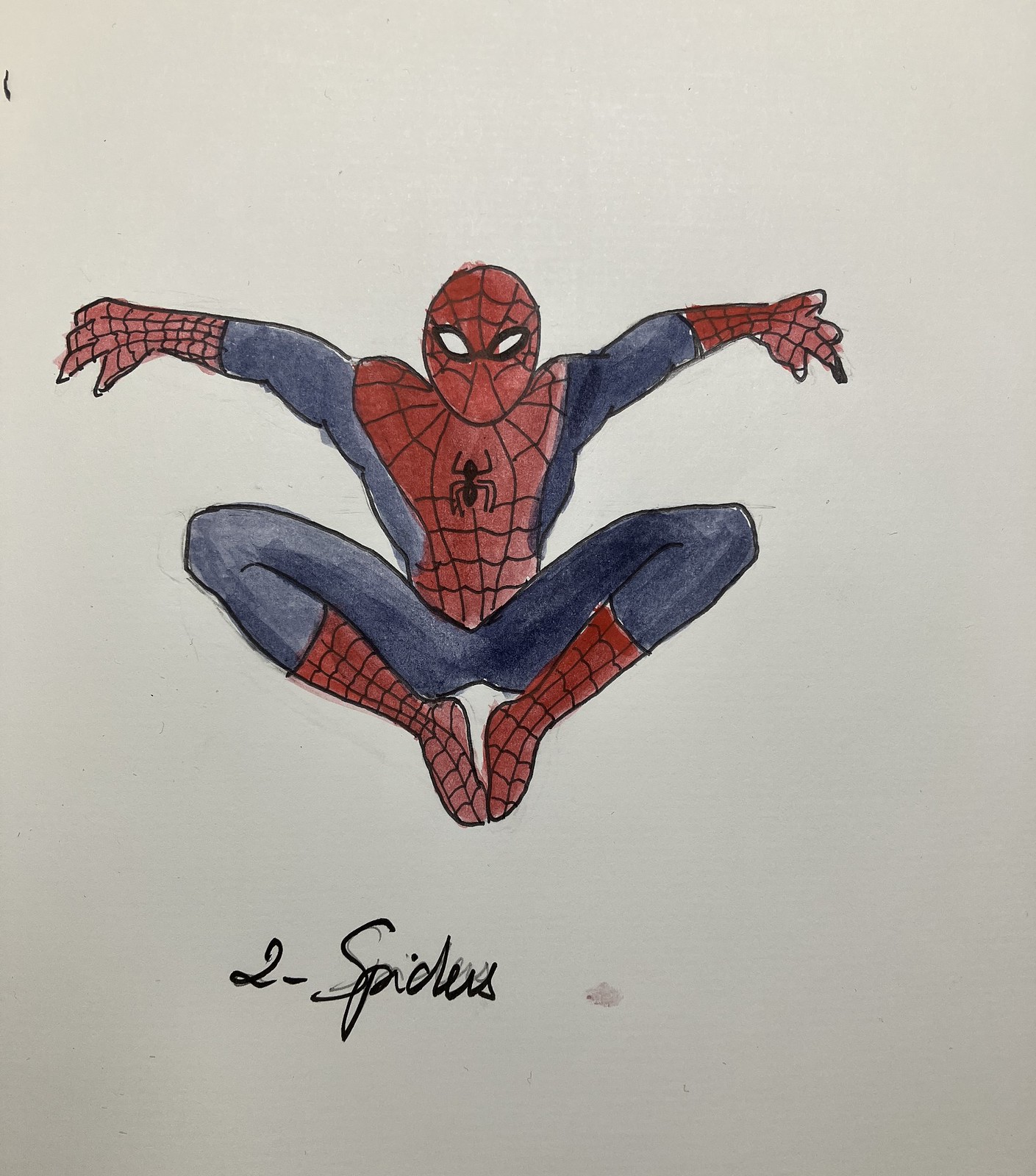This drawing depicts Spider-Man, meticulously colored with colored pencils, set against a backdrop of very light gray paper. Below the illustration, in black ink, is the notation "2 - Spiders." Spider-Man is portrayed facing the viewer, with his arms extended behind him and his knees drawn up towards his chest, his feet near the top of his thighs. His iconic costume is vividly detailed, featuring red gloves and boots that resemble spider webs. His full-face mask mirrors this web-like pattern, with large white eyes outlined in black. The web design continues across his chest and shoulders, where a black spider emblem is prominently displayed.